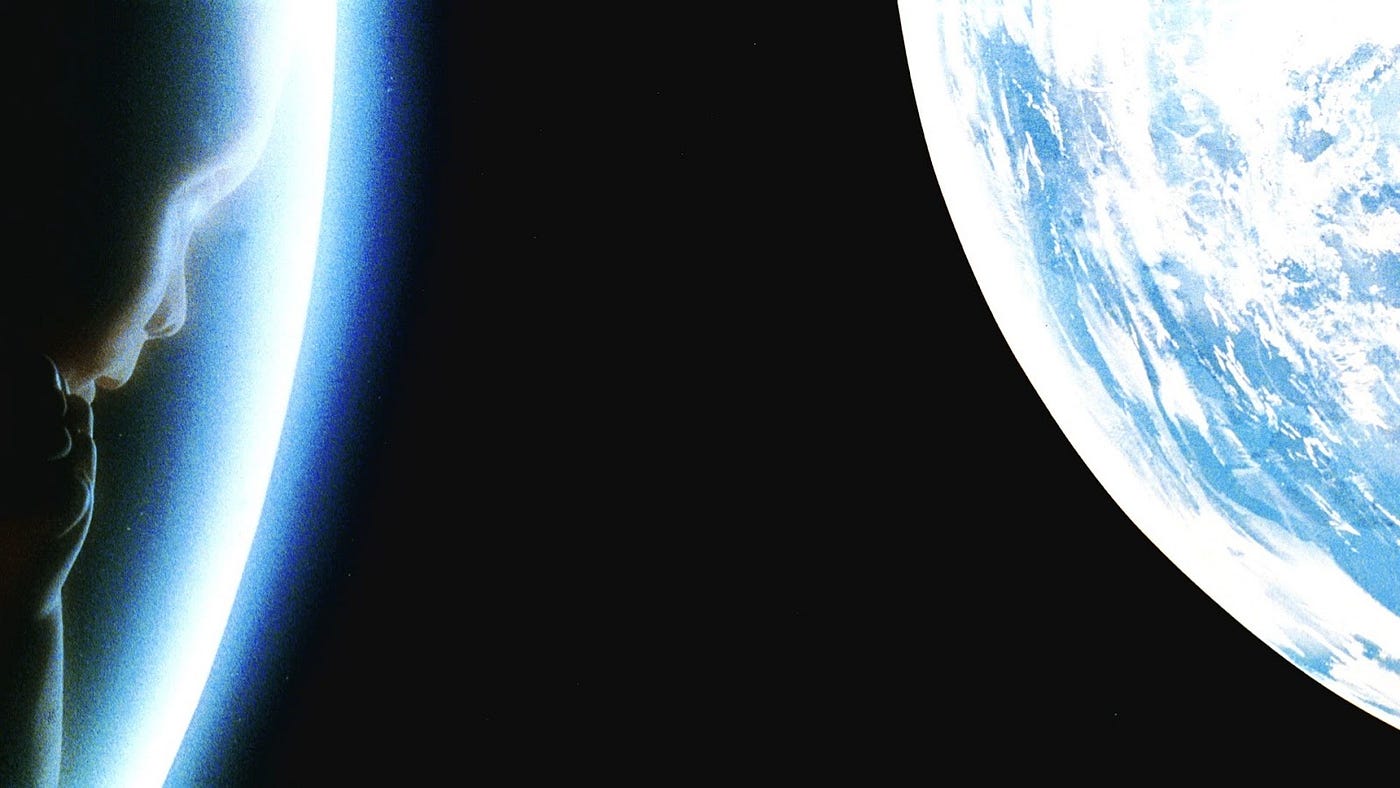The image appears to be a highly detailed and evocative depiction of outer space, featuring elements that evoke both the celestial and the human. On the right side, there is a striking view of roughly a quarter of the Earth, characterized by its deep blue hues and scattered white clouds, set against the vast backdrop of jet-black space. In stark contrast, on the far left side of the image, emerges a silhouette of a young child, most likely an unborn baby. This delicate figure, seeming to peer downwards from the upper left corner, is marked by a subtle touch of light— a white glimmer in its eye, a cream-colored nose, and its lips slightly parted. The baby’s hand gently touches beneath its chin, contributing to an introspective posture.

Separating the Earth and the child, a glowing blue streak of light cuts through the darkness, anchoring from the top downwards slightly to the left. This streak is brightest at the center, fading gradually to a darker blue at the edges. The space behind the child is almost entirely black, creating a profound contrast that highlights the luminescent qualities of the blue line and the gentle features of the silhouette. Together, these elements weave a narrative that spans the infinite vastness of space and the intimate quietude of human life.